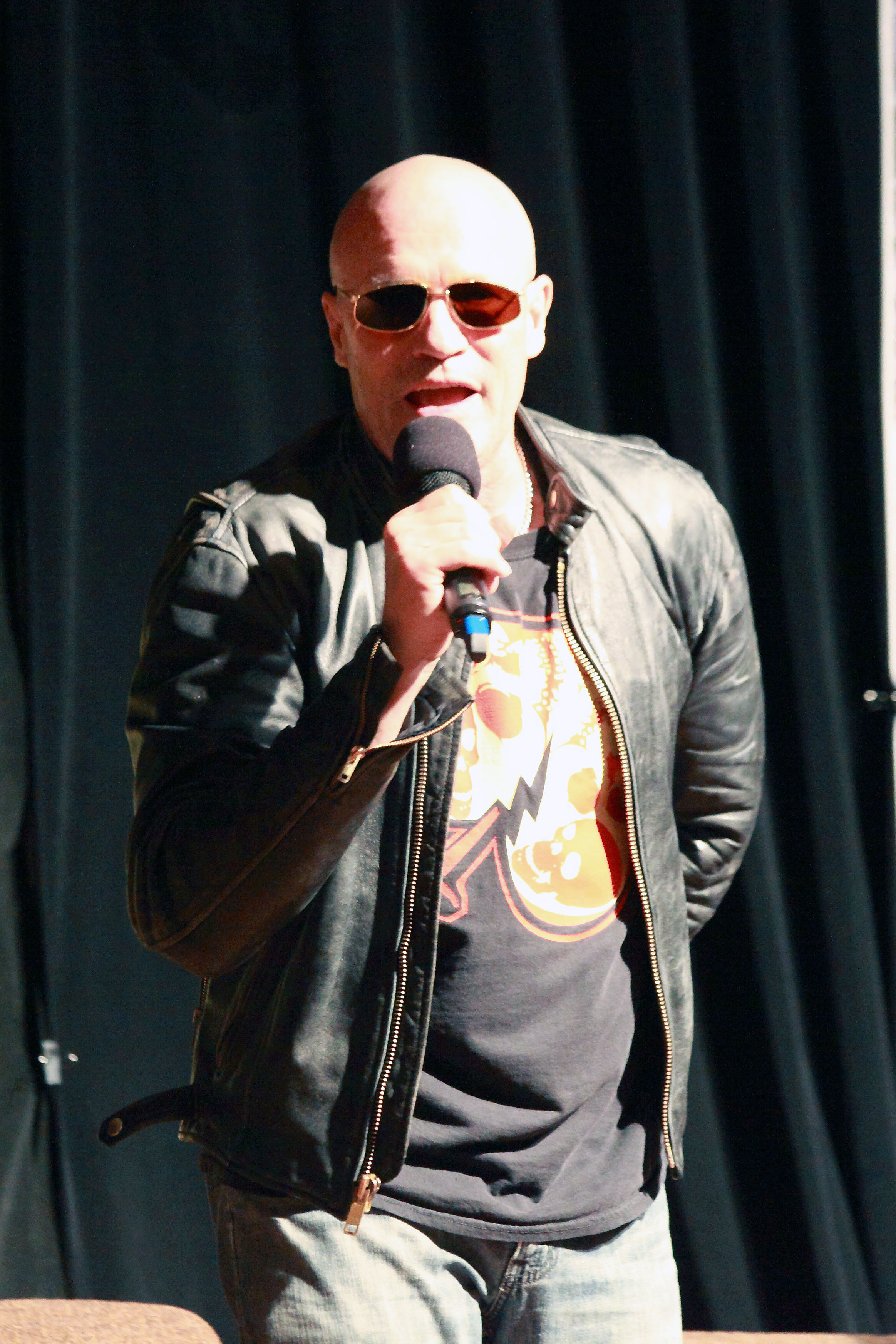This photograph features a man with a bald head, standing and speaking into a black microphone with a rounded end. He is wearing gold-rimmed sunglasses with brown reflective lenses, a black graphic t-shirt with an orange skull design, and faded blue jeans. His black leather jacket, which is worn and features gold zippers on the sleeves and front, is open. The man’s left hand is positioned behind his back while his right hand holds the microphone close to his mouth, which is open as he speaks. The setting appears to be illuminated by a strong, bright light coming from the right side, casting distinct shadows. The background is dominated by a black curtain wall with several ripples in the fabric, held up by black paper clips. In the bottom left corner of the image, there is a glimpse of a tan fabric chair, hinting that it may have been part of the staging, along with a visible metal piece. Overall, the man exudes a confident presence, likely addressing an audience, with the black curtain providing a stark backdrop to emphasize his figure.